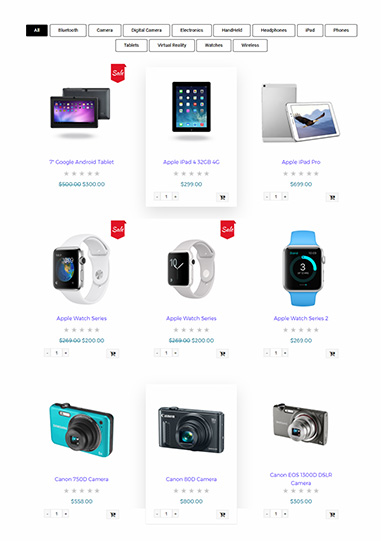This vertical rectangular image showcases a detailed catalog layout with a variety of electronic products arranged neatly on a webpage.

At the very top of the image, there is a row of small horizontal rectangular buttons. Each button contains a word in black font. The first button reads "All" and stands out with white lettering on a black background. The remaining buttons each have white backgrounds, black lettering, and black outlines, making it challenging to decipher the text due to the small size. The third button reads "Camera" and the fourth reads "Digital Camera," while the others are largely illegible.

Below these navigation buttons, there is another row of four centered buttons, similar in style to the ones above.

The main section of the image is organized into three rows of product images, with three products in each row.

- **First Row**:
  - The first product is a tablet with a "Sale" tag in white on a red background at the upper right corner. Below the image, in purple text, it reads "7-inch Google Android tablet," with the price listed in green.
  - The second product appears to be an iPad. Underneath, in purple text, it says "Apple iPad," but the remaining details are hard to read. The price is displayed in green below the description.
  - The third product is a white iPad labeled "Apple iPad Pro" in purple text, with the price also in green.

- **Second Row**:
  - The first item is an Apple Watch with a white band. The purple text below the watch reads "Apple Watch Series," followed by the price in green. This watch also has a "Sale" tag.
  - The second item is another Apple Watch with a light gray band, also labeled "Apple Watch Series" with the price in green and a "Sale" tag at the corner.
  - The third watch in this row is labeled "Apple Watch Series 2" with a bright blue strap, and the price is indicated in green below the image.

- **Third Row**:
  - The first item is a teal-colored Canon camera. The text reads "Canon" followed by an unreadable model number, with the price displayed in green.
  - The second camera is black and labeled "Canon," possibly reading "800 camera," with the price in green.
  - The third item is another type of camera, with the specifics not clearly readable.

The structured layout visually communicates the diversity and pricing of each product, though some text is difficult to decipher due to the small font size.